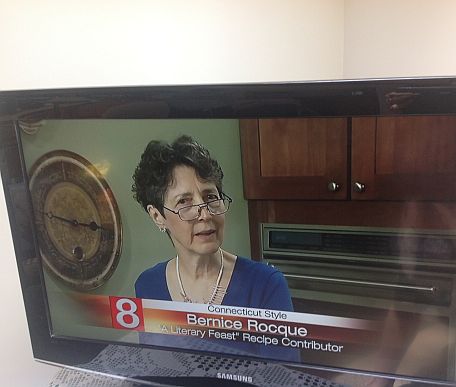In this detailed color photograph, we are gazing at a small Samsung screen, which could be either a television or a computer monitor, set in the corner of a room with beige walls. The screen, resting on a white doily, is noticeably tilted so that the left side is further away than the right. Positioned towards the bottom right corner of the image, the screen mainly displays content from Channel 8 news.

On the screen, we see a woman with short dark hair and glasses, dressed in a blue V-neck shirt and wearing a necklace. She stands in her kitchen, which is discernible by the brown wooden cabinets and a stove with metallic handles behind her. The kitchen wall, contrasting with the room's beige walls, is painted a vibrant lime green. An elaborate clock hangs on this green wall to her left. Additionally, a graphic banner at the bottom of the screen reads "8, Connecticut Style, Bernice Roke, a Literary Feast Recipe Contributor," adding context to the image with its colorful array of text and backgrounds in black, brown, green, red, orange, yellow, and white.